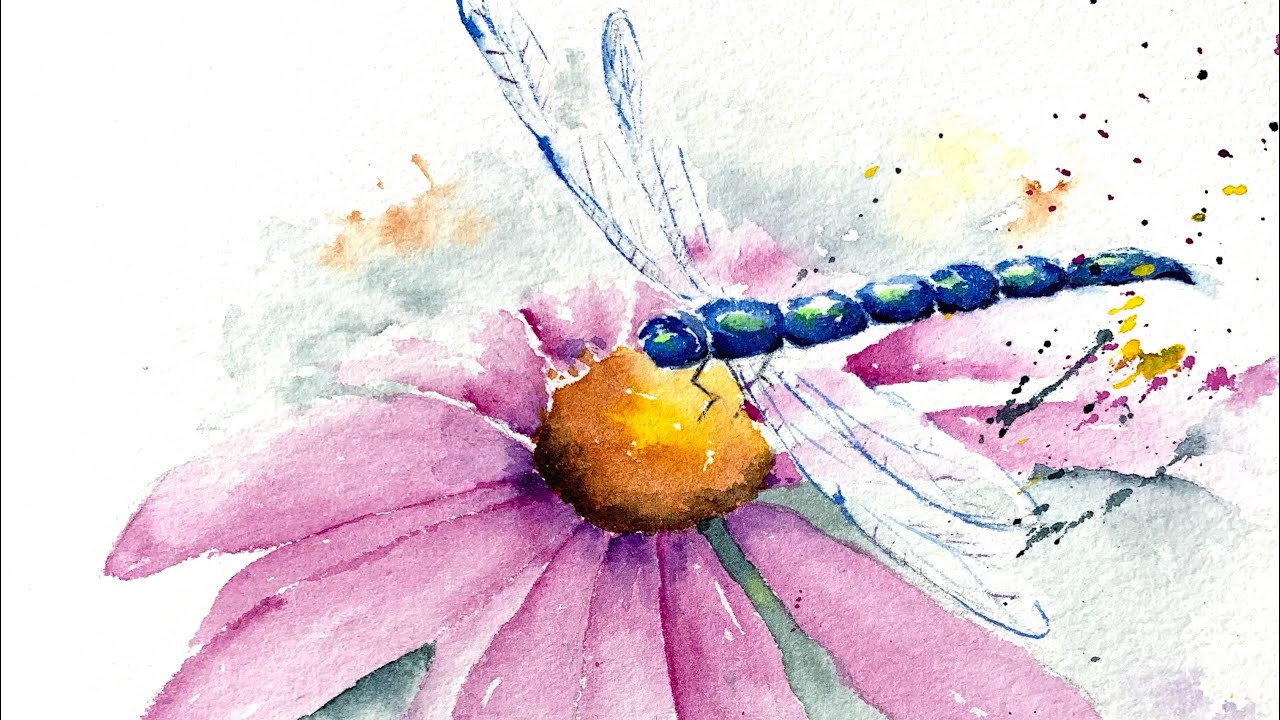The painting depicts a detailed floral scene set against a solid white background. Central to the artwork is a vibrant flower with a yellow center surrounded by delicate pink petals. Just beneath the pink petals, green leaves provide a touch of natural contrast. A blue dragonfly, characterized by its translucent white wings—two pointing upwards and two downwards—rests delicately on the flower. The dragonfly's body, segmented into seven parts including the head and tail, is adorned with green dots. Adding an abstract element to the scene, random paint splatters are particularly noticeable in the upper right corner of the canvas.